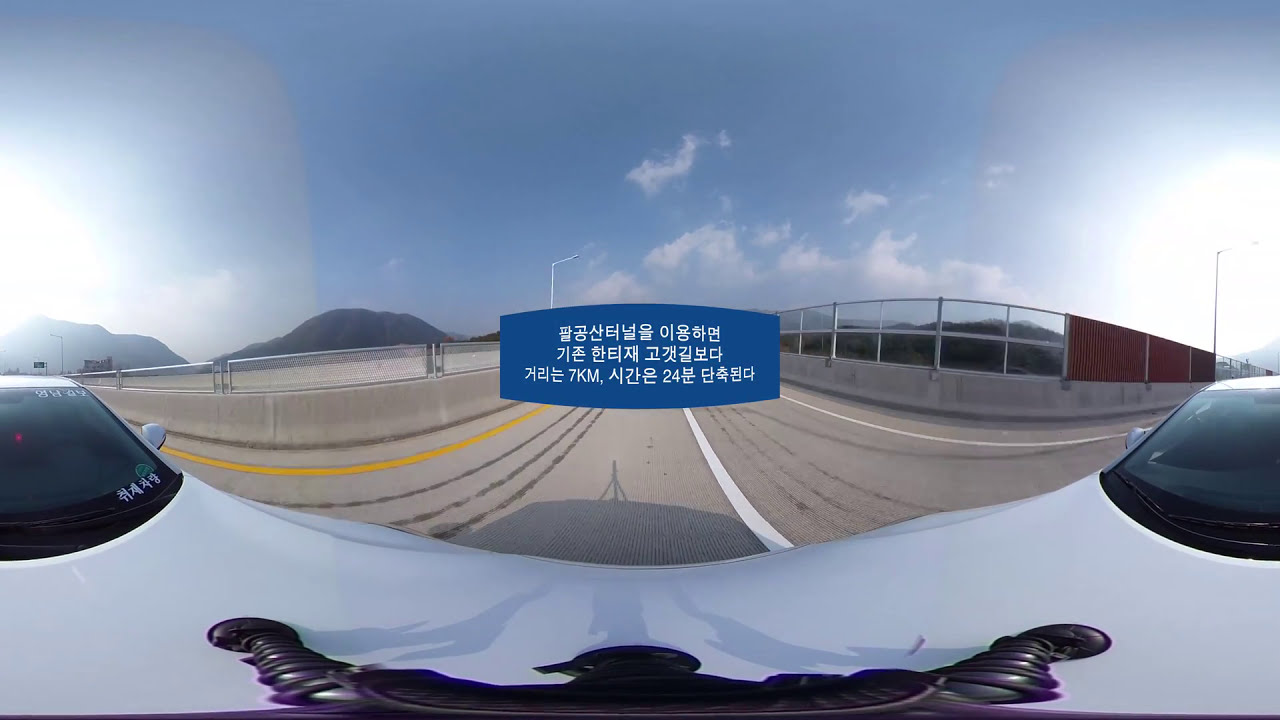This image captures a daytime scene on a highway or bridge, depicted with a convex lens effect that curves the surroundings. A white vehicle is prominently featured in the image, but the lens distortion creates the illusion of two joined cars. The car's black windshields and side mirror are clearly visible. Surrounding the vehicle are yellow and white lane markings on the gray road surface. The highway is flanked by concrete barriers with fencing atop them, and there is a silver railing attached to a reddish-orange wall to the right. The left side features a gray cement wall with a silver gate above it. 

A blue box with white text, possibly in Korean or Chinese, is centrally located on the image. The text includes "7 kilometers" and "24," and an image of a human figure resembling a superhero with raised hands is also noted. The background reveals a blue sky with wispy, feathery clouds and distant mountain ranges that have a bluish hue. Sunlight illuminates the scene, enhancing the vivid colors of the sky and the landscape.